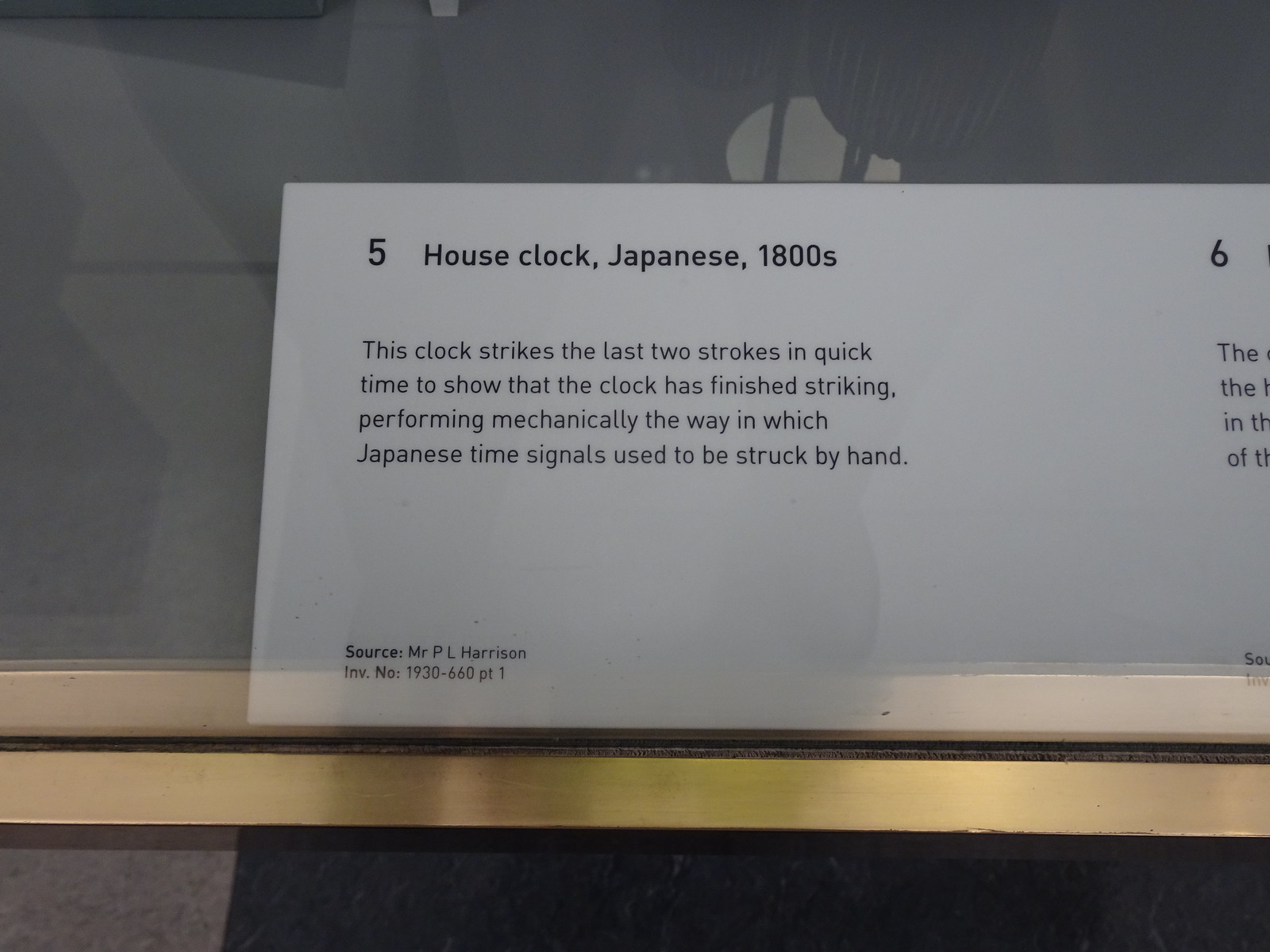The image shows a museum placard, predominantly white, set against a gray background with gold trim. The placard features the text "No. 5, House Clock, Japanese, 1800s." Below this title is a detailed description reading, "This clock strikes the last two strokes in quick time to show that the clock has finished striking, performing mechanically the way in which Japanese time signals used to be struck by hand." At the bottom left corner, the placard credits "Source: Mr. P. L. Harrison, INV.NO 1930-660PT 1." The background around the placard varies in shades of gray, and adjacent to it appears another placard labeled "No. 6" with a different description, though this is not the focus of the image. The house clock itself is not visible in the image; only the informational placard is shown.